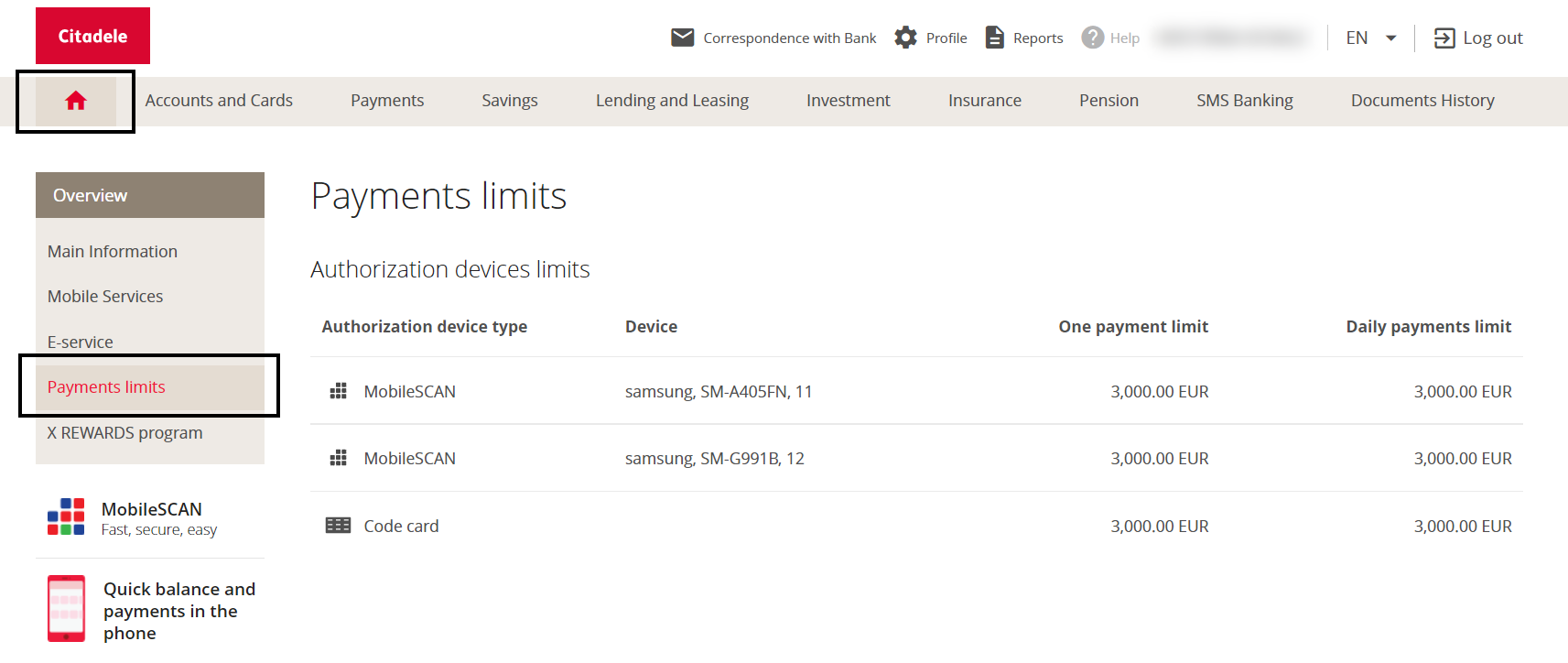In the top-left corner of the image, the word "CITADEL" is prominently displayed in white text against a rich red background. Adjacent to this, on the far right side, is a vertical column of tabs featuring the options: correspondence with bank, profile, report, help, and language (currently set to English), followed by a logout button in the top-right corner. The majority of the background is a clean white, providing a stark contrast.

Directly below the "CITADEL" label on the left side, there is a red home button outlined by a black square. To its right, a panel lists several tabs, including: accounts and cards, payments, savings, lending and leasing, investment, insurance, pension, SMS banking, and document history.

On the left side of this panel, underneath the "CITADEL" title, there is a section labeled offer human and a subsequent list featuring: mail information, mobile services, e-services, payment limit (which is currently selected and highlighted in red with a black outline), and the X reward program. Below this menu, there is an overview section that states: "Mobile scan, fast, secure and easy," followed by "Quick balance and payment on the phone," with a corresponding picture of a red phone.

The right side of the image is dedicated to the main page display, which currently shows details about the "payment limit" section highlighted on the overview. It features the title "Payment Limit" and further elaborates with "Authorization device limit" below. A detailed table spans three rows and four columns, outlining specific authorizations and limits. The first column, labeled "Authorization device type," lists "Mobile scan" and "Code cut." The second column, "Device," specifies "Samsung SMA0405FN11" for the first mobile scan, and "Samsung SMG991B12" for the second. The third column, "Online payment limit," and the fourth column, "Daily payment limit," both show consistent limits of €3,000 for each device and code cut authorization method.